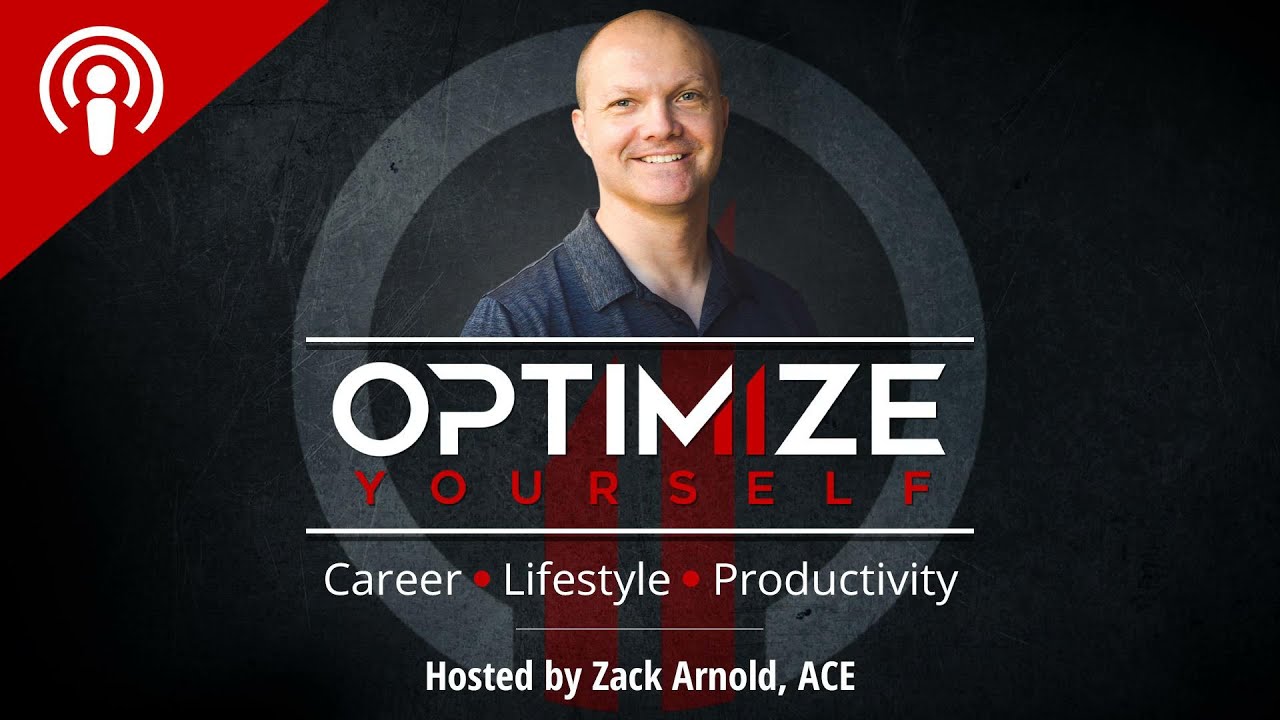The image is an advertisement for the "Optimize Yourself" audio podcast, hosted by Zach Arnold, ACE. At the center is a smiling Caucasian man in his 30s or early 40s, with short hair, nearly bald, wearing a gray polo shirt. The background features a gray circular design with red decorative elements resembling an equal sign. Prominently displayed in the middle is the text "Optimize Yourself" in red and white. Below it, the words "Career, Lifestyle, Productivity" are listed in white, each preceded by a red bullet point. The image also contains a graphical audio icon in the upper left corner, which includes a white head silhouette and a red triangle, indicating audio signal strength. Further down, it states "Hosted by Zach Arnold, ACE" in white lettering.